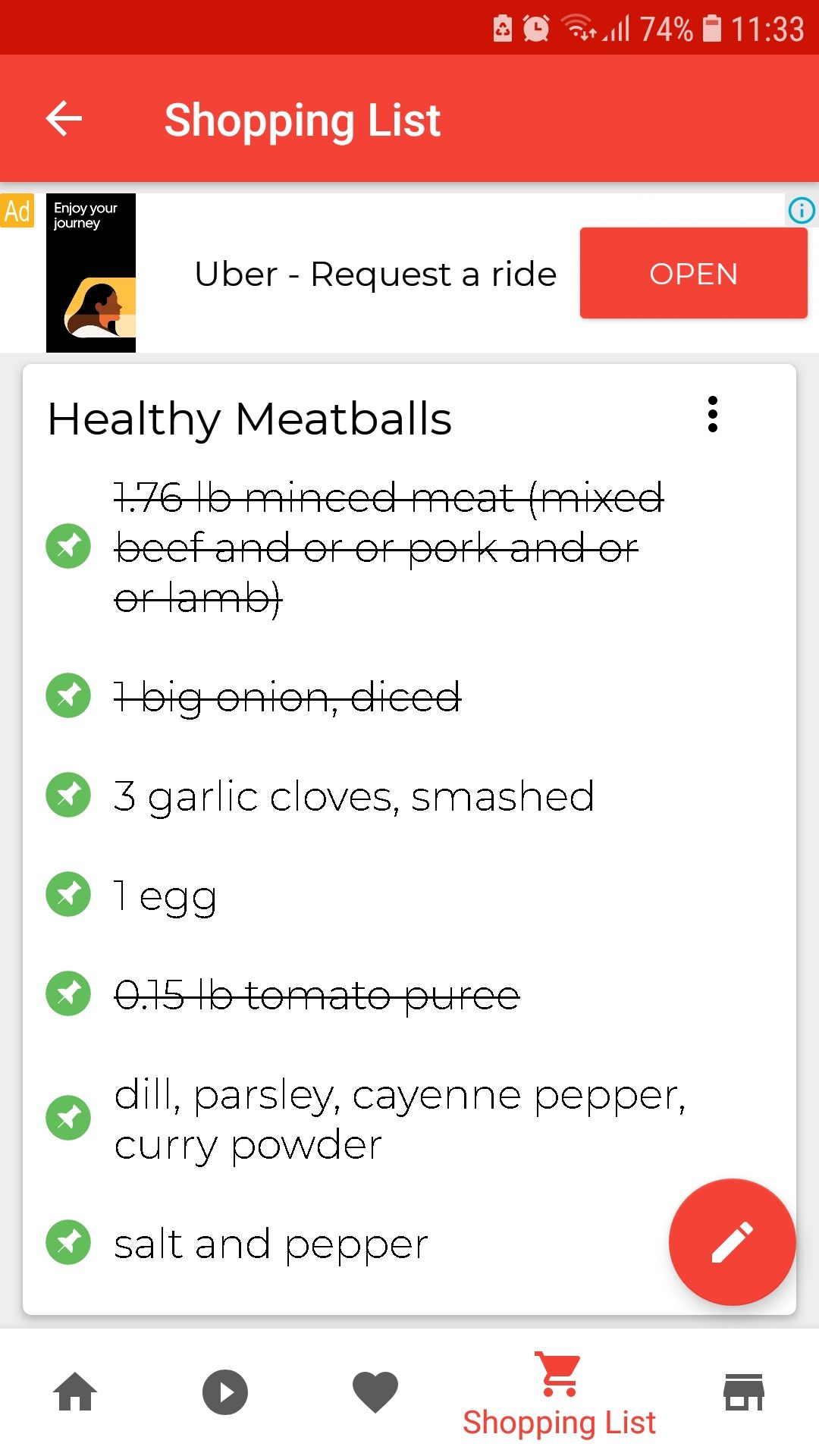This image captures a screenshot of a digital shopping list interface. At the top right corner, there are several icons alongside a battery indicator showing 74% and a time display reading 11:33. The upper section of the screen features a dark red banner, transitioning to a lighter red banner below. In bold white text, the title "Shopping List" is displayed with a leftward-pointing arrow situated on the leftmost side.

Beneath this banner, there's a yellow box with the label "Add" in white font. Adjacent to it, an icon promoting Uber's "Request a Ride" service is set within a red rectangle bearing the word "OPEN" in bold white caps. Below this, a white rectangular box with black text highlights the list item "Healthy Meatballs" and is accompanied by a three-dot menu icon on the right.

The main portion of the list itemizes various groceries, each prefixed by a green circle enclosing a white thumbtack icon. Here's the detailed inventory:

1. 1.76 pounds minced meat (mixed beef, pork, or lamb) - crossed out
2. One bag onion, diced - crossed out
3. Three garlic cloves, smashed
4. One egg
5. 0.15 pounds tomato puree - crossed out
6. Dill
7. Parsley
8. Cayenne pepper
9. Curry powder
10. Salt and pepper

Four items—garlic cloves, egg, dill, parsley, cayenne pepper, curry powder, and salt and pepper—remain unchecked, while three items have been crossed out, indicating they have been acquired.